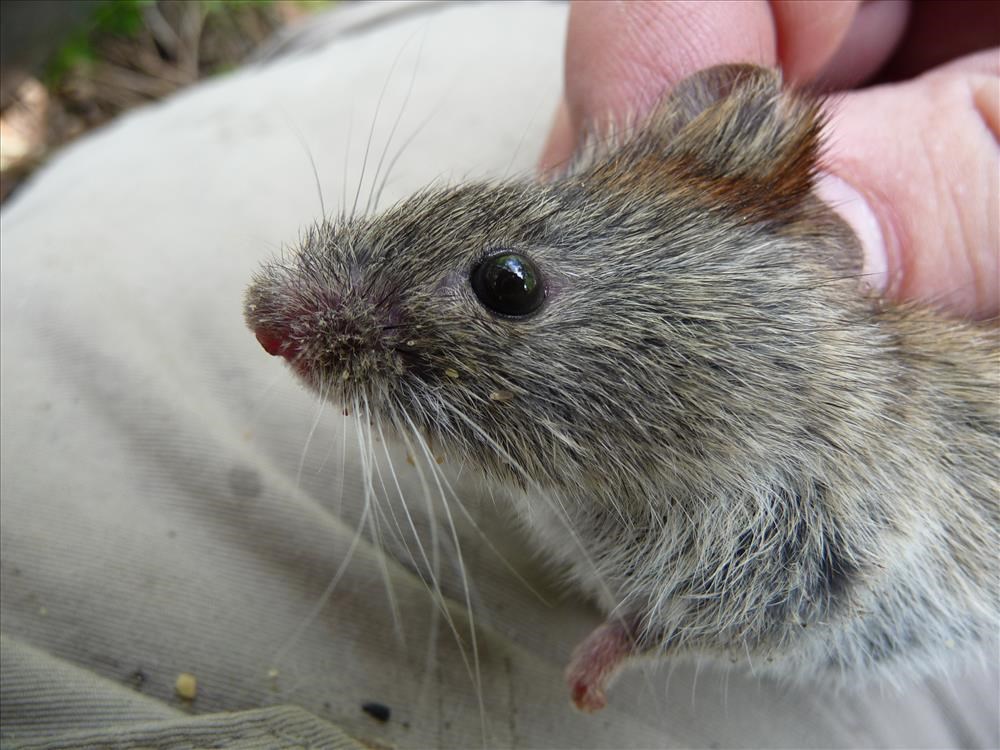This detailed close-up photograph captures the front half of a small gray rodent, likely a mouse or a rat, with a few white patches amidst its predominantly gray fur. The rodent has a prominent black, beady eye and large, white whiskers extending from its pink nose. Its slightly browner ears and pink paws are also visible. The animal appears to have food crumbs around its mouth. 

A light-skinned human hand, likely male, is holding the rodent by the scruff of its neck, using the thumb and index finger. The background includes the person’s beige or white pants and the outdoors, with a green bush and plant roots visible in the upper left corner. The positioning and details strongly indicate the rodent is being held outside.